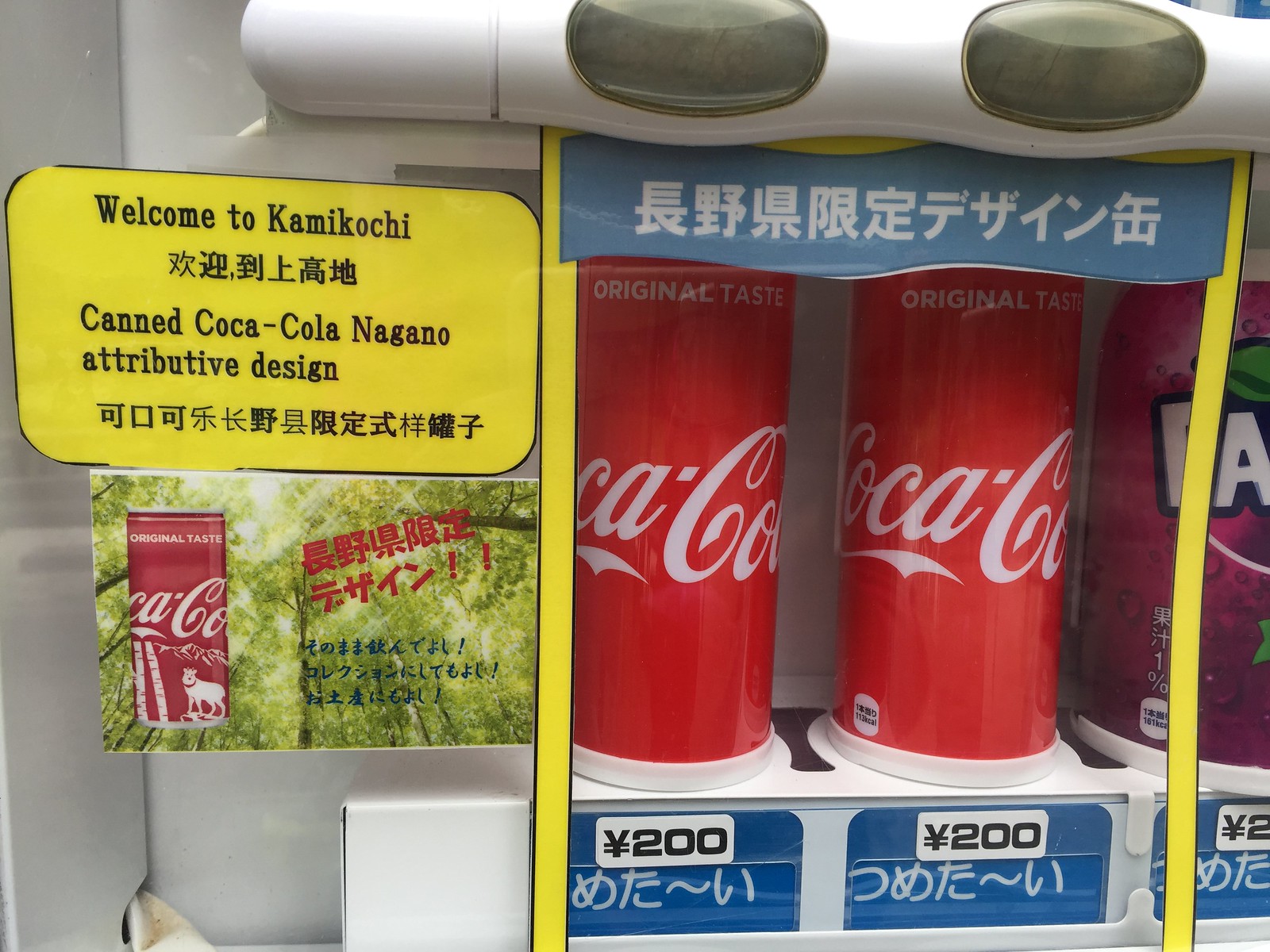This photograph captures a close-up of a vending machine situated in Japan. Prominently displayed in the machine are two red cans of Coca-Cola, featuring the iconic white "Coca-Cola" script through the middle and the phrase "Original Taste" at the top of each can. The price for the Coca-Cola is listed as 200 yen. To the left side of the vending machine is a yellow sticker with black lettering that reads, "Welcome to Kamakochi." Below this, the text continues with, "Canned Coca-Cola Nagano Attributive Design," accompanied by more Asian lettering. Adjacent to the sticker is an image of a Coca-Cola can, along with red and blue Asian text, set against a background of a tree canopy with sunlight filtering through. On the right side of the image, a partial view of another beverage, likely a grape Fanta, is visible.